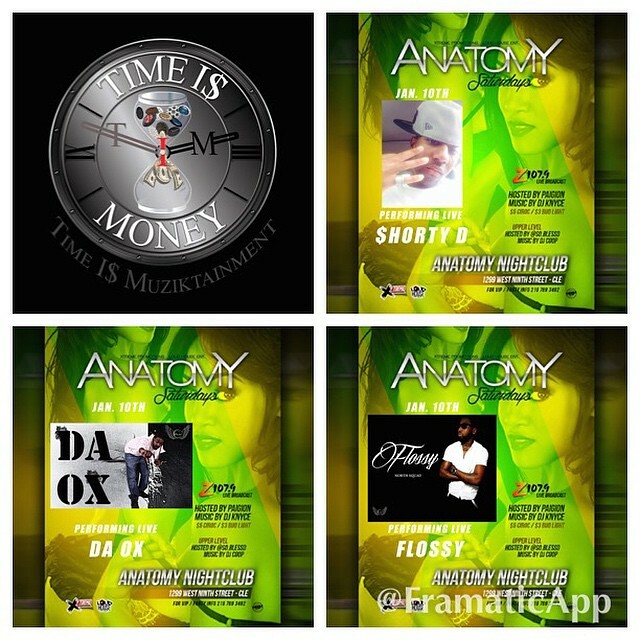The image is a composite of four distinct but related advertisements, arranged in a two-by-two grid format. The top left quadrant features a visually striking time-themed graphic: a clock with a silver face and black hands, overlayed by an hourglass with buttons or beads trickling down and transforming into dollar bills. The phrases "Time is Money" (with the 'S' in 'is' stylized as a dollar sign) and "Time is Musictainment" are emblazoned across the design. The other three quadrants function as promotional flyers for an event called Anatomy Saturdays at Anatomy Nightclub, likely sponsored by Z107.9. Each flyer showcases January 10th as the event date, and features vibrant lime green and yellow backgrounds with images of beautiful women. Prominent African-American performers are highlighted, with names like Shorty D, the Ox, and Flossie, each identified as performing live. A watermark from the 'Attic App' at the bottom of the collective image hints at its likely creation over a decade ago.